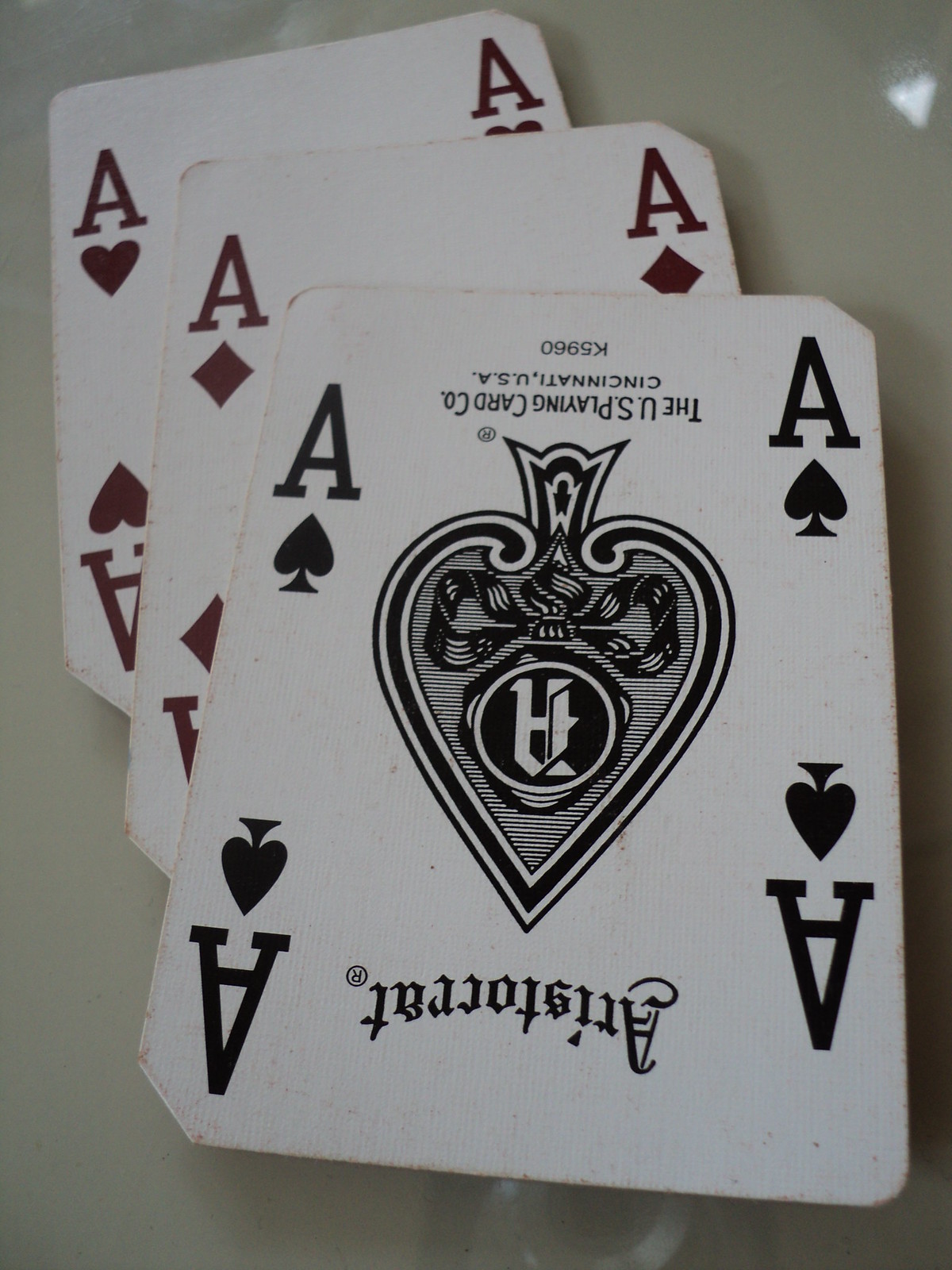A set of playing cards is arranged on a highly polished, light gray surface, either a table or a counter. The surface's sheen reflects light, giving it a shiny appearance. The cards, predominantly white, are all aces and are presented in a layered, slightly spread out manner, revealing the presence of three individual cards. The top card, positioned upside down, is the black ace of spades and bears the brand name "Aristocrat" along with "The U.S. Playing Card Company, Cincinnati, USA, K-5-9-6-0." The middle card is the red ace of diamonds, and the bottom card is the red ace of hearts.